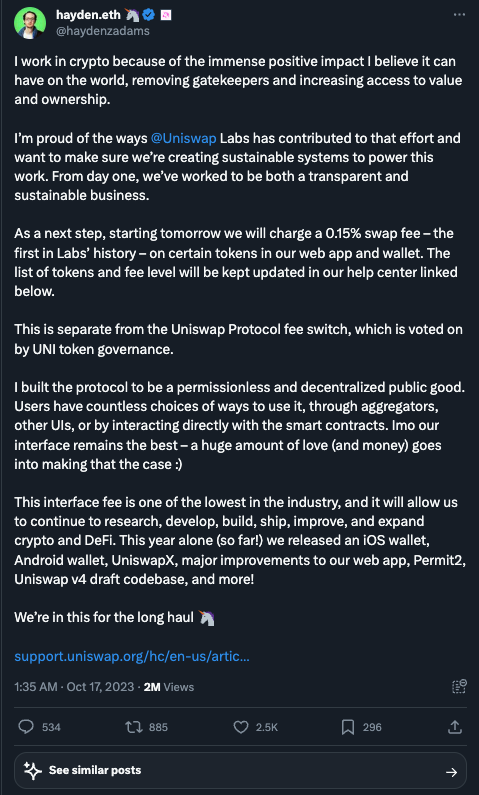The background of the image features a dark navy blue or possibly a very dark blackish-blue color, creating a deep, muted ambiance. Centered in the foreground is a profile picture set against a green background. The person depicted is not clearly visible, making their features indistinguishable. They appear to be wearing a blue and white shirt that has writing in white displaying "Hayden.ETF" alongside a grayish unicorn icon. 

Adjacent to the unicorn, there is a bluish circle with a check mark, indicating verification, and a white box containing a pink element that is not clearly visible. The username "@Hayden C Adams" is displayed nearby.

A detailed text overlay exists in the image, organized in several paragraphs. The first reads:
"I work in crypto because of the immersive positive impact I believe it can have on the world by removing gatekeepers and increasing access to value ownership. I'm proud of the ways @Uniswap Labs has contributed to the effort and want to ensure we're creating sustainable systems to power this work. From day one, we've aimed to be both transparent and sustainable businesses."

The next paragraph outlines a forthcoming change:
"As a next step, starting tomorrow, we will charge a 0.15% swap fee—the first in labs’ history—on certain tokens in our web app and wallet. The list of tokens and fee levels will be updated regularly, and I will link more details below."

A subsequent section clarifies:
"This fee is separate from the Uniswap protocol fee switch, which is voted on by UNI token governance."

Further text elaborates on the protocol's ethos:
"I built the protocol to be a permissionless, decentralized public good. Users have countless ways to engage, whether by aggregating through other UIs or interacting directly with the smart contracts. Although many interfaces are available, our I/O interface remains the best thanks to an enormous amount of love, effort, and community support."

Concluding with a call to action, the text states:
"Support us at uniswap.org/hc/en-us/art."

At the bottom of the image, displayed in white text, is the timestamp "1:35 AM, October 17th," accompanied by a view count that indicates the message has been seen over 3.2 million times.